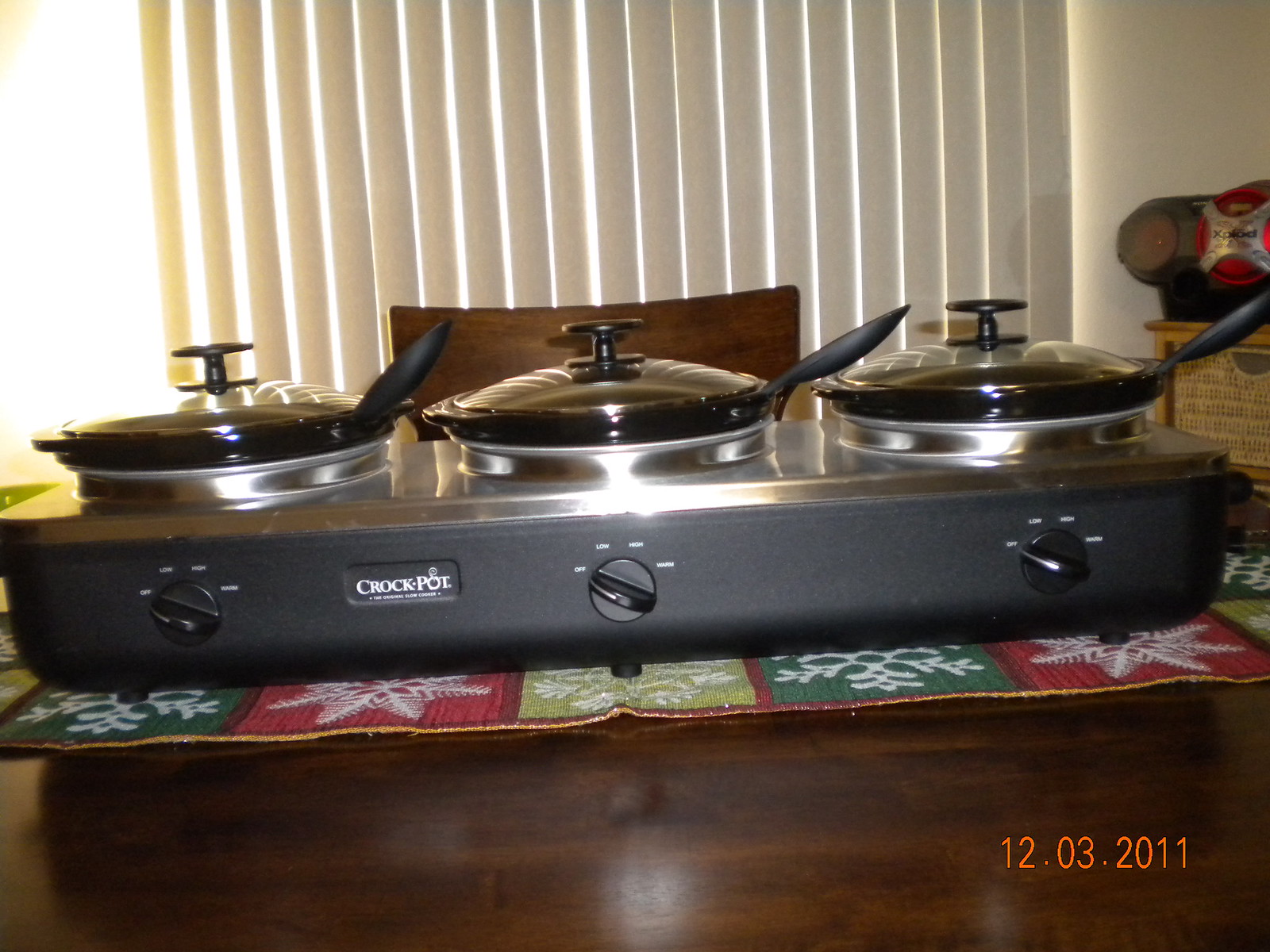This photograph, dated 12-03-2011, showcases a multi-unit Crock-Pot buffet server, prominently set on a wooden kitchen table adorned with a festive placemat featuring snowflakes and a Christmas motif pattern. The device, sporting a blackish gray body with chrome accents, consists of three individual crock pots each equipped with their own heating elements and round glass lids. Each pot is securely nestled within its designated container area and features dials at the front with four temperature settings: off, low, high, and a single line indication. The Crock-Pot logo is clearly visible on the front of the unit. In the background, a wooden chair is partially visible behind vertical blinds that block out external light, and a small wicker and wooden shelving unit stands to the right, enhancing the domestic ambiance of the scene.